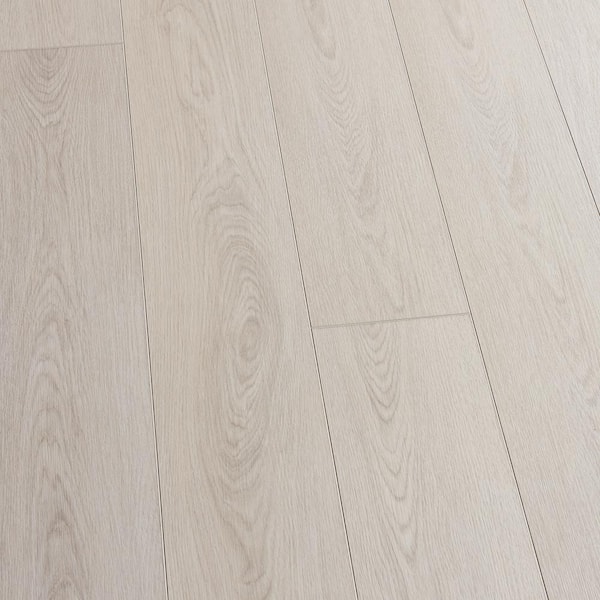This rectangular, portrait-oriented image presents a top-down view of a floor crafted from wood planks or a similar wood-like material. The flooring comprises five distinct rows of planks running diagonally from the bottom center towards the upper left. Each plank reveals intricate wood grain patterns, some featuring knots while others exhibit purely linear grain details. Two rows include horizontal joints where shorter planks are adjoined: one joint is situated on the far left in the upper section, and another is positioned centrally but closer to the right-hand side.